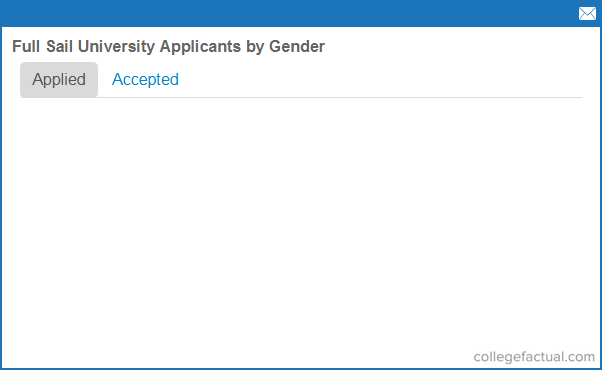This screenshot depicts a webpage with a predominantly white background, featuring a prominent blue banner and a greenish-blue border along the bottom and side. In the upper right corner, there is an envelope icon, suggesting it might be related to a mail application. Along the top of the window, the text reads "Full Sail University Applicants by Gender." Below this heading are two distinct tabs labeled "Applied" and "Accepted." In the lower right corner, the source of the webpage is identified as "collegefactual.com." The overall design is minimalistic, with a clean layout and specific data categories related to university applicants displayed for users.